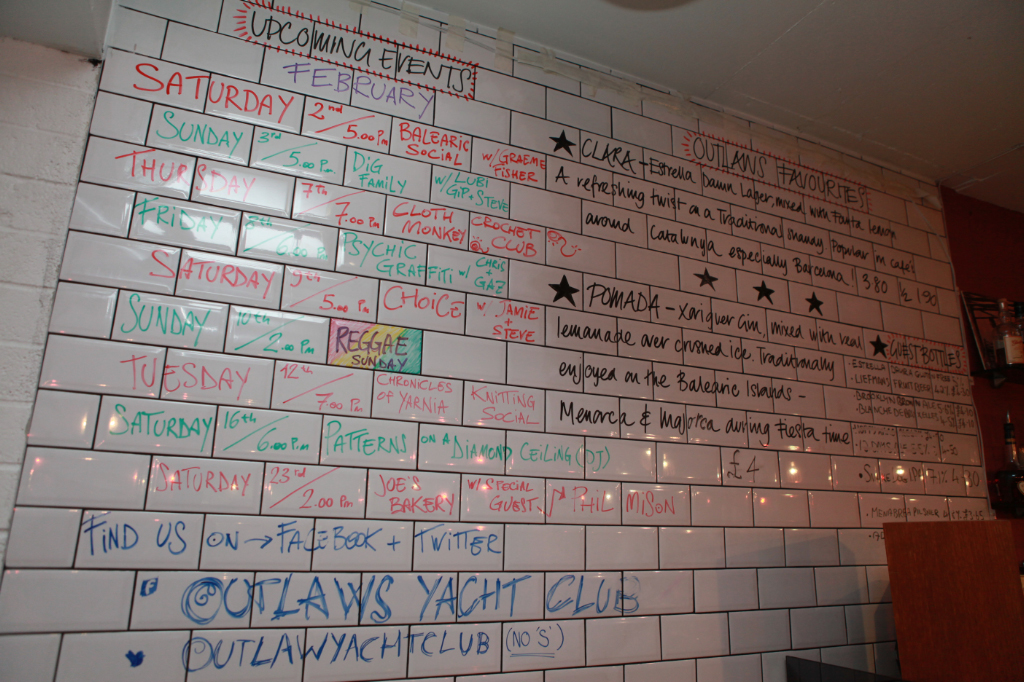The image depicts a white, glossy tiled wall resembling white bricks, covered with text written in markers of various colors. The wall is viewed at an angle, allowing visibility of both the left and right sections. On the left side, there is a heading, "Upcoming Events, February," followed by a list of events in red and green markers for different days of the week, detailing times and activities like "Balearic Social with Graeme Fisher" on Saturday, 2nd at 5pm. On the right side, the text reads "Outlaw's Favorites" in black marker, listing several names, some of which have stars next to them, such as Clara and Pomada. Additionally, there is a section labeled "Guest Bottles" and multiple references at the bottom left corner that encourage finding the venue on social media under "Outlaw Yacht Club."